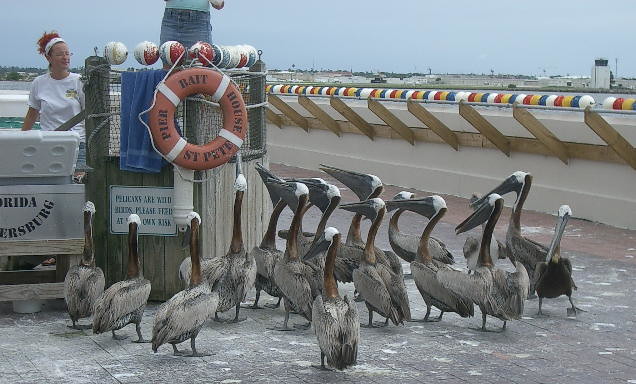In this vibrant image, approximately 12 to 16 adult brown pelicans are clustered on a wooden boardwalk by the ocean, their presence transforming the tranquil pier into a bustling scene. Each pelican boasts a distinctive appearance with gray bodies, brown necks adorned with dark black spots, white heads, and elongated black beaks complemented by a prominent black throat pouch. The birds stand attentively, facing a person on a raised platform, mysteriously cropped at the top, who appears to be the source of their intense gazes, likely awaiting scraps of fish bait. 

The platform features a conspicuous orange buoy inscribed with "Pier Bait House St. Pete" in black text and is situated next to a large white cooler brimming with fish bait. Additionally, a woman with red hair stands nearby the cooler, participating in the feeding routine. The background, under a bright blue sky, reveals glimpses of sandy beach and distant buildings. The boardwalk itself, worn to a gray hue, is littered with bird droppings, further illustrating the pelicans' frequent visits. Decorative buoy-like balls in various colors line the railing, adding maritime charm to this lively coastal scene.